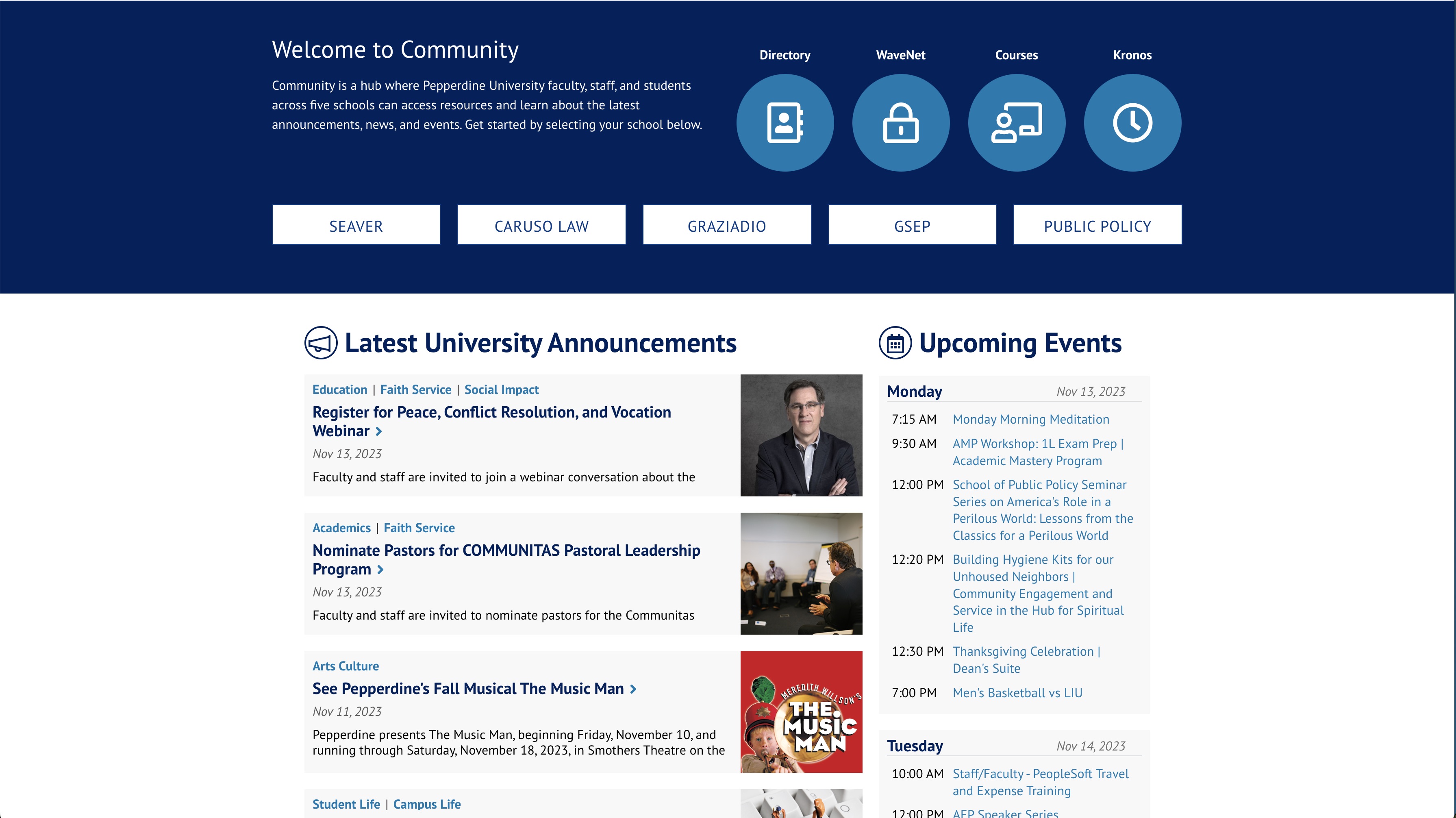The image features a structured layout of various sections and elements. At the top, the background is a dark blue with the words "Welcome to Community" displayed prominently in white. Below this, the word "Directory" appears, accompanied by a blue circle. Further down, there is another blue circle displaying the image of a person near a blackboard. Beneath these, several white squares list choices labeled "SEAVER," "Caruso Law," "GRAZIADID," "GSEP," and "Public Policy."

On the left side, there is an area featuring a circular icon of a megaphone, labeled "Latest University Announcements." To the right, a similar circular icon shows a calendar, labeled "Upcoming Events." 

In the center top of the image, there is a picture of a man in a suit with dark glasses, set against a dark gray background. Directly below this, another image shows people seated around a conference table.

At the bottom, the background color shifts to red, with the text "The Music Man" prominently displayed. Next to this text, there is a small image of a man holding either a telephone or a maraca, though the small size makes it difficult to identify clearly.